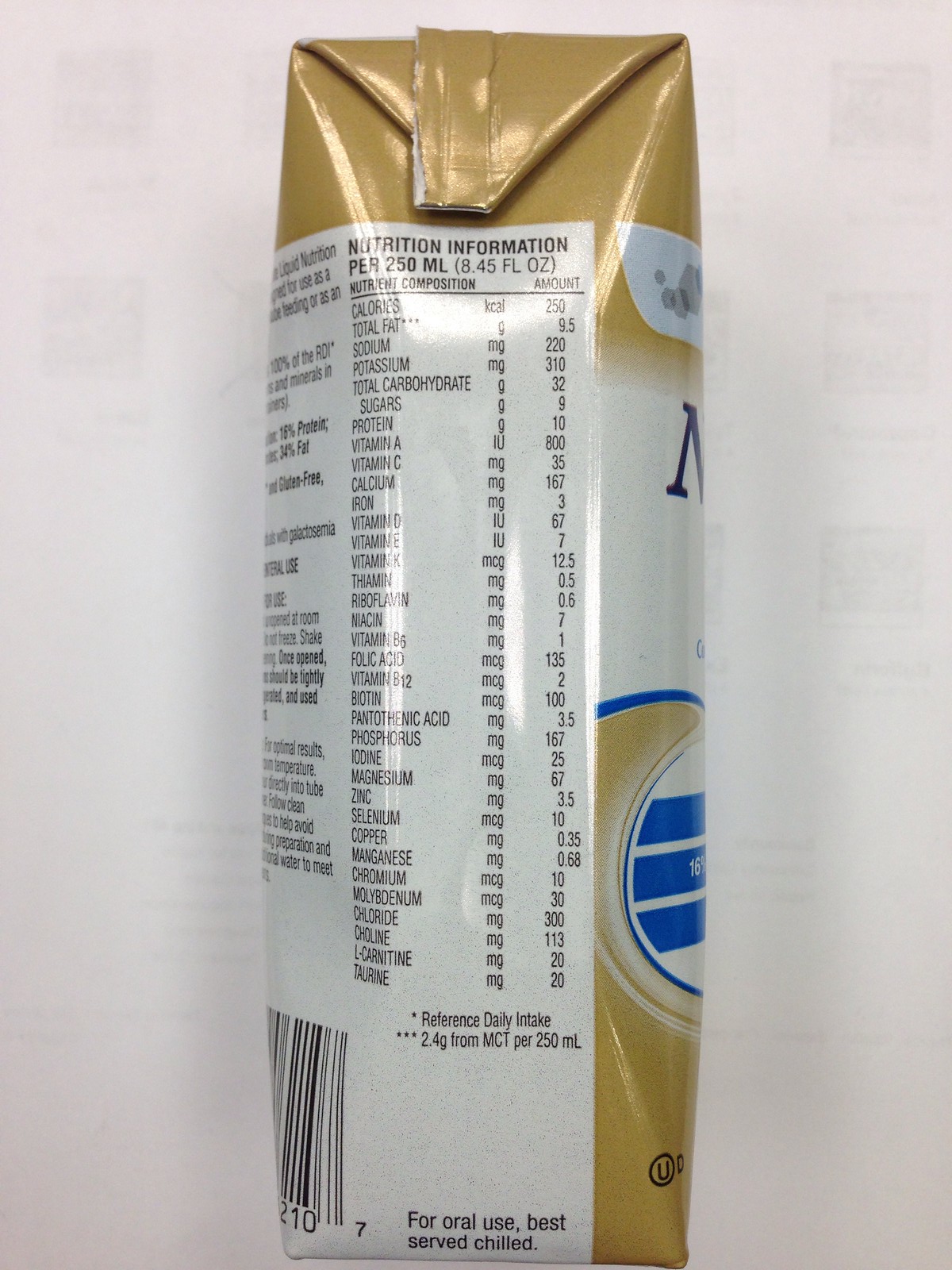This photograph features a drink carton set against a white background. The carton, primarily gold at the top and transitioning to white in the middle, has visible creases and crinkles, suggesting it's made from cardboard. It prominently showcases a dark blue logo on the side. The photo captures the side of the carton that displays comprehensive nutritional information in a black font on a white section, listing calories, fat, sodium, potassium, and other nutritional stats. Additional details are found on the back of the packaging, including the ingredient list, more facts, and a barcode positioned at the bottom. Instructions reading "for oral use, best served chilled" are also visible at the bottom, emphasizing the intended way to consume the beverage.